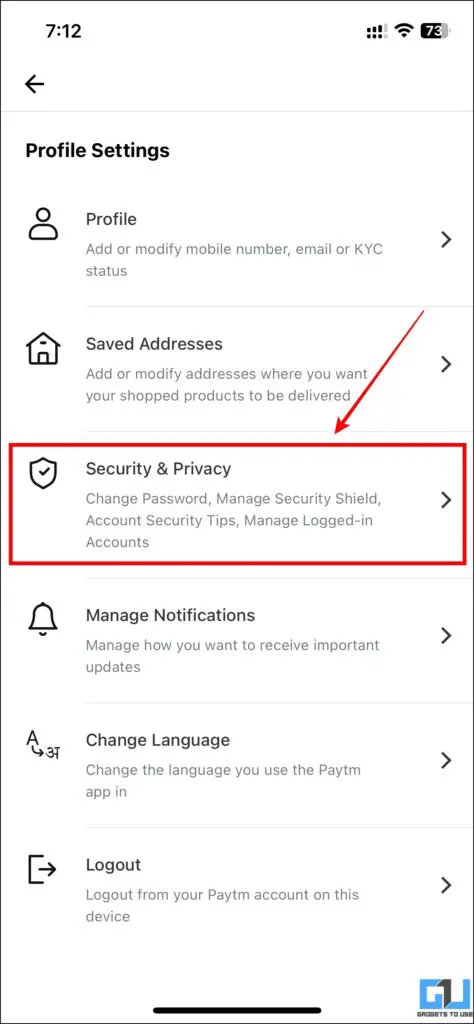The image features a black notebook and a tablet providing a detailed interface related to user profile settings. The tablet screen displays various options, including the ability to add or modify mobile numbers and email addresses, check accuracy status, and handle full billing and security addresses. There are prompts to add or modify delivery addresses for shot buttons. A red arrow points to screen privacy settings, followed by a shield icon labeled "Change Password" to manage security measures. Further options include account security tips and managing locked accounts, as well as notifications settings to control how important updates are received. There is a section for changing the app's language, indicated by a square icon, and a logout option for the Paytm account on the device. The bottom of the screen shows different sections in blue and black, typifying the app's distinctive organizational scheme.